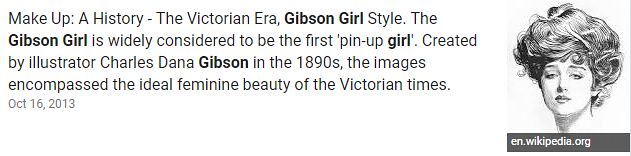The image features a detailed section of text on a white background, left-aligned, titled in black, "Makeup: A History - The Victorian Era Gibson Girl Style," where "Gibson Girl" is emphasized in bold. The main paragraph informs us that the "Gibson Girl," again bolded, is widely considered to be the first pin-up girl, a term where "girl" is also bolded. This iconic figure was created by illustrator Charles Dana Gibson in the 1890s and represented the ideal feminine beauty of the Victorian era. Below this paragraph, in smaller text, is the date, "October 16, 2013," still left-aligned. 

To the right of this textual content is a square, black-and-white drawing of a woman with an elaborate, dark hairstyle. Her hair is styled tall and curls elegantly around the edges, pinned up in a striking Victorian fashion. The woman appears youthful and seems to gaze off thoughtfully. Beneath this image is the URL "en.wikipedia.org," suggesting that the excerpt originates from Wikipedia.